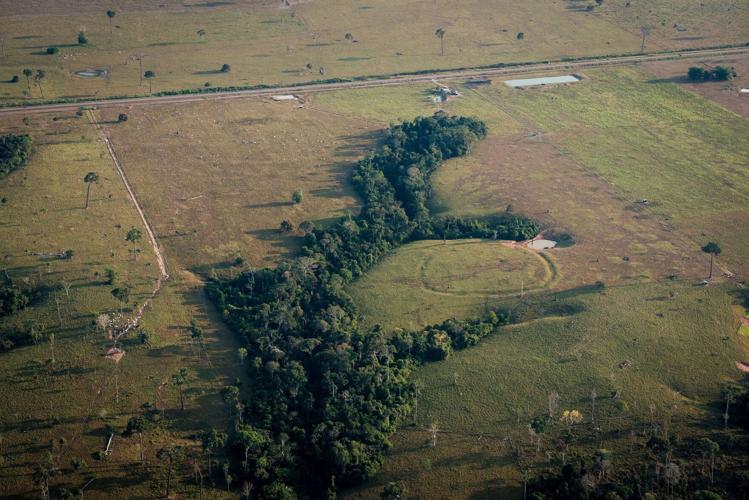An aerial view captures a vast, flat landscape dominated by vibrant green grass and intricate tree lines that meander whimsically across the scene, almost resembling an animal reclining. At the heart of this natural tapestry lies a distinct circular formation, its edges meticulously mowed, creating noticeable indentations into the ground. Surrounding this enigmatic circle, the dark green foliage of the tree lines starkly contrasts with the lighter grass, all under a clear sky with no visible structures like houses or barns. The panorama is further enriched by distant roads and possible sand pits, adding to the intrigue of this seemingly serene yet mysterious expanse.